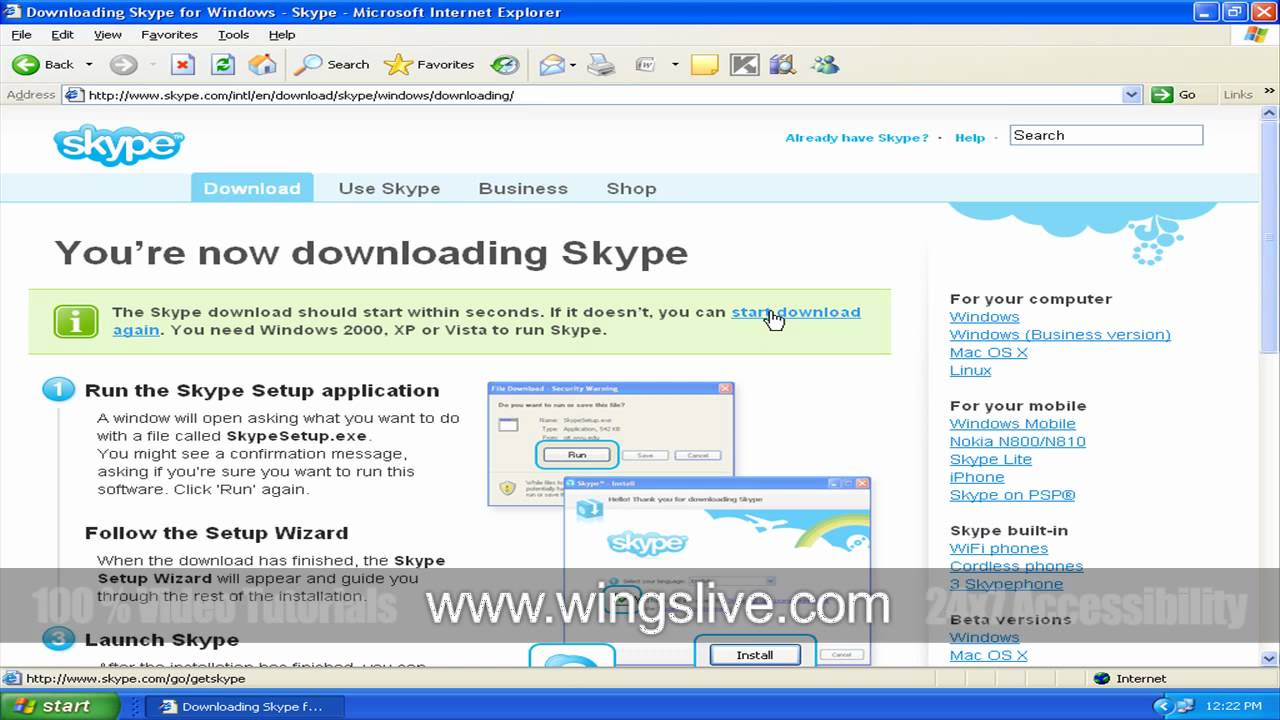The website image displays the process of downloading Skype for Windows using Internet Explorer. At the top, a blue banner prominently suggests downloading Skype, while just below it appears the familiar file menu bar with options such as File, Edit, and View. The webpage itself, hosted on Skype.com, features several navigation tabs: Skype, Download, Use Skype, Business, and Shop, with additional options for 'Already Have Skype', 'Help', and 'Search'.

A message on the page indicates that the Skype download will start automatically, advising users to restart the download via a provided button if it doesn't initiate within seconds. Compatibility requirements are specified: Windows 2000, XP, or Vista for older systems, as well as alternative versions for Mac OS X and Linux, and various mobile platforms.

Detailed steps for installation are outlined: running the Skype setup application, dealing with potential confirmation prompts for running the software, and following further setup instructions. A gray banner at the bottom of the screen includes the URL www.wingslive.com, amidst the scrolling text of installation guidance.